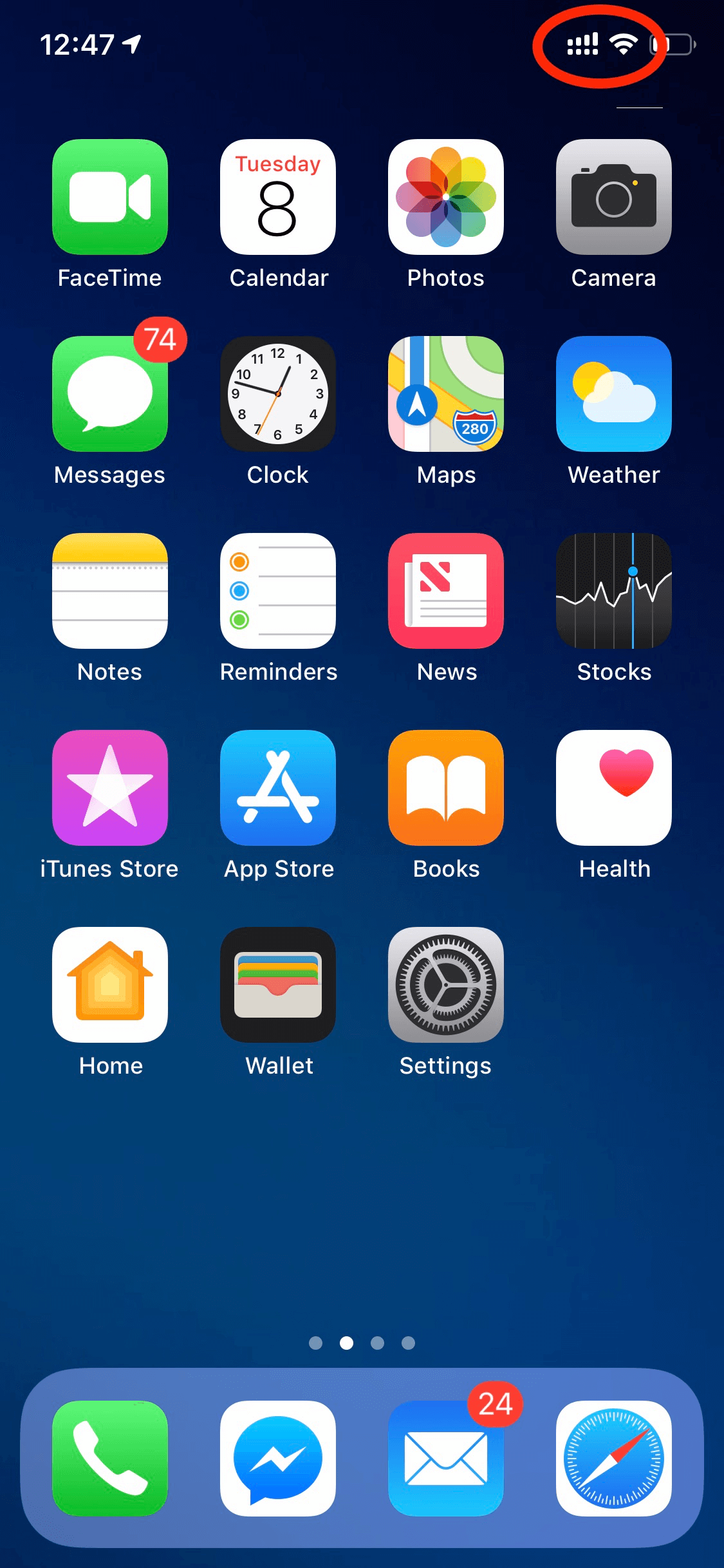The image showcases the home screen of an iPhone, filled primarily with default application icons. These include FaceTime, Calendar, Photos, Camera, Messages, Clock, Maps, Weather, Notes, Reminders, News, iTunes Store, App Store, Books, Health, Home, Wallet, and Settings. The dock at the bottom of the screen features frequently used apps: Phone, an alternative messaging app, Mail, and Safari. Notably, the Mail app displays a badge with 24 unread messages, and the Messages app shows a badge with 74 unread messages.

In the top-right corner of the screen, the notification area is highlighted by a red circle or oval that has been edited into the image. This is done to draw attention to the unusual cell reception indicator, which, instead of showing the typical bars, uses a series of exclamation points. These exclamation points increase in size, mimicking the progression of a normal signal strength display.